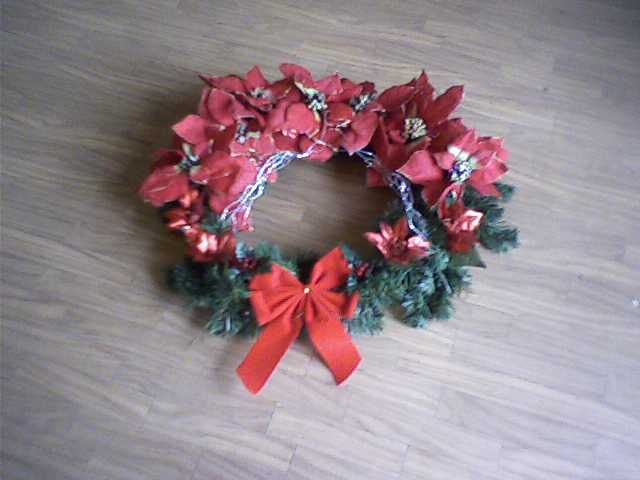This photograph captures a festive Christmas wreath set against a light brown and gray wooden floor marked with subtle lines. The wreath boasts a traditional round shape, made up of green pine needles predominantly visible towards the bottom and peeking out from the sides. The top two-thirds of the wreath is adorned with vibrant red flowers, likely poinsettias, their petals interspersed with tiny white centers and potentially small red berries. At the very bottom of the wreath, a red ribbon cinched with a small silver, almost yellow pinpoint adds a finishing touch. Wisps of white material can be seen wrapping through parts of the wreath, possibly binding the decorations together. Overall, the image provides a festive and visually rich display, though some details appear slightly blurred.